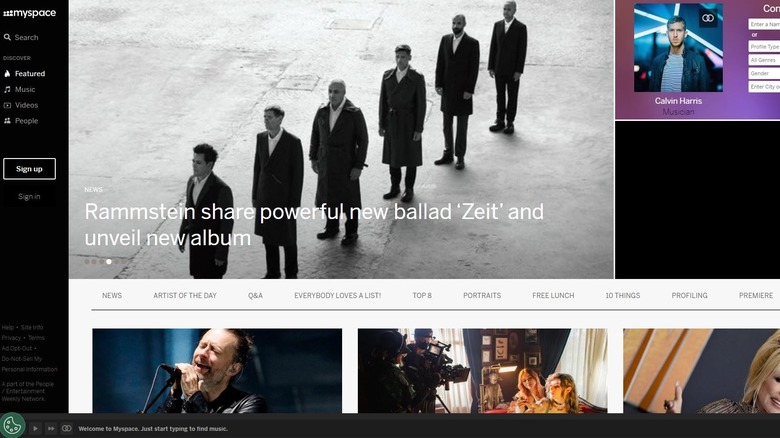The image is a screen capture of the MySpace online application. Prominently displayed in the upper left is a black-and-white photograph of six men standing in a diagonal line, each dressed in black jackets and coats over white shirts, paired with dark-colored pants. Superimposed across the bottom of this photograph in white text are the German words "Rammstein," "Scher," "Powerful," "New Ballad," "Sitz," and "Unveil New Album."

Below this main image, there are three smaller images aligned horizontally in a row. The first image on the left captures a close-up of a man singing into a microphone, showing his head and shoulders. The middle image features a group of people operating movie cameras, directing the equipment toward two women. The third and final image on the right shows a partial close-up of a female performer, capturing just half of her face.